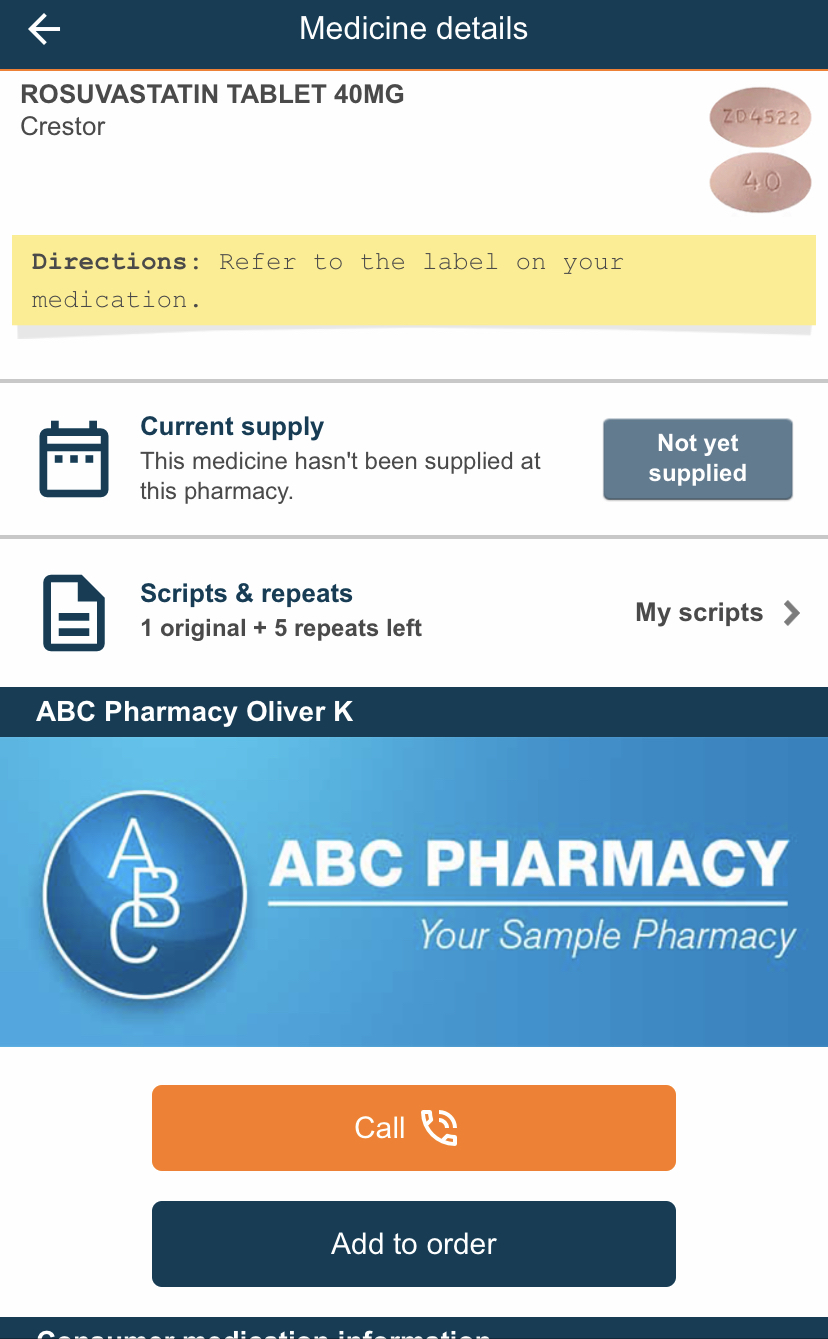The image depicts a user interface of a prescription website for medication. In the upper left-hand corner, a left-pointing arrow icon indicates the option to navigate back to the previous page. Centered at the top of the screen is the heading "Medicine Details." Directly beneath this heading, the medication is identified as "Rosuvastatin tablet, 40 milligrams," with the name spelled out as "R-O-S-U-V-A-S-T-A-T-I-N." Adjacent to this text on the right is an image of a pill labeled "ZD4522." Below this, the brand name "Crestor" is displayed alongside another pill image imprinted with "40."

Further down, the section titled "Directions" advises users to refer to the label on their medication for specific instructions. Underneath, a status update labeled "Current Supply" indicates that this medication has not been supplied at the pharmacy in question, marked on the right with "Not yet supplied." A horizontal gray line divides this section from what lies beneath.

Below the divider, a segment titled "Scripts and Repeats" informs the user that they have "One original plus five repeats left" on this prescription, with an option on the right labeled "My Scripts." Centrally positioned on the screen is the name of the pharmacy, "ABC Pharmacy, Oliver K.," accompanied by an image of the pharmacy, labeled again as "ABC Pharmacy" or "Sample Pharmacy."

At the bottom of the interface, two action buttons are visible: a "Call" option highlighted in orange, and, immediately below it, an "Add to Order" button.